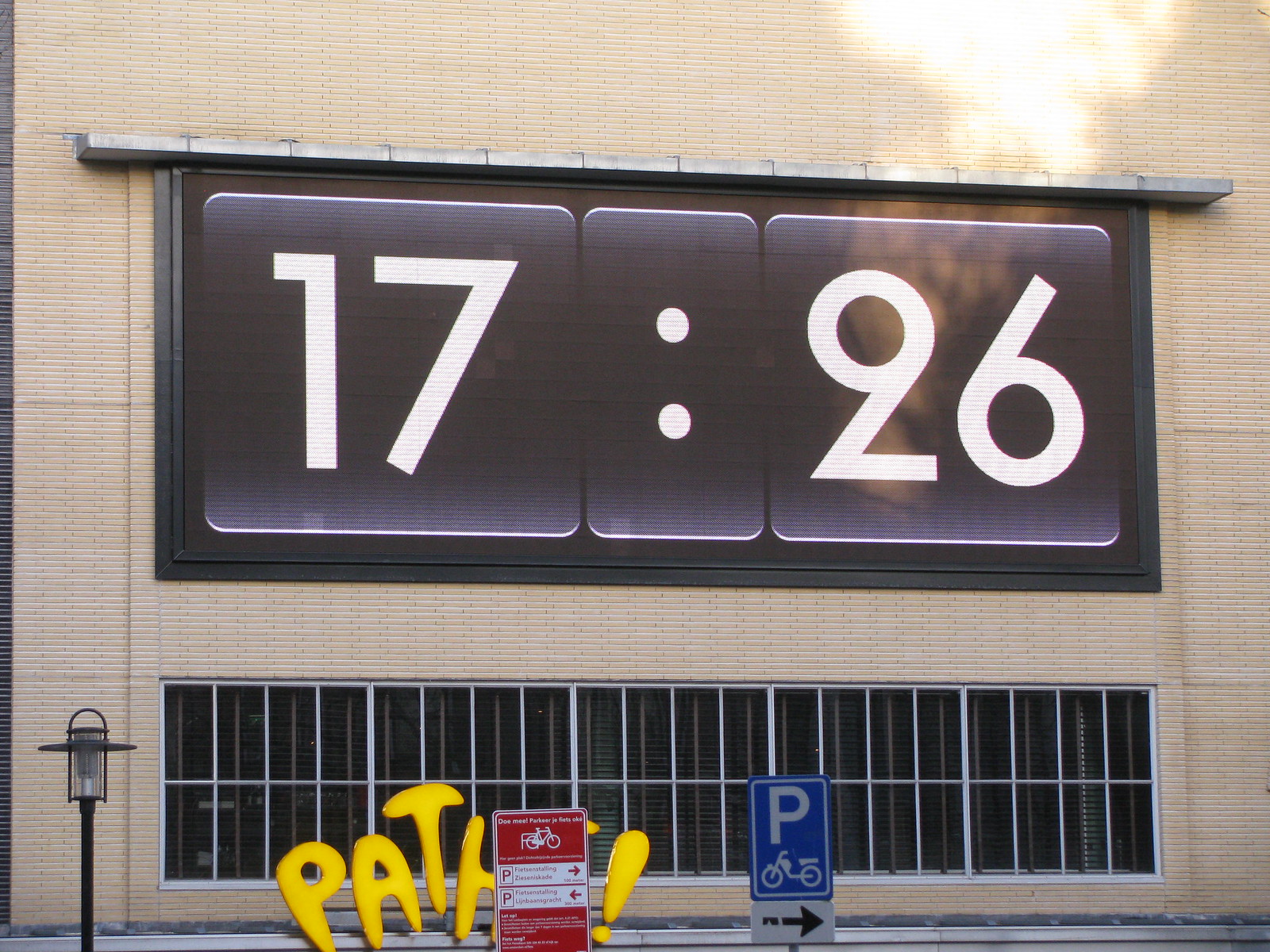This photograph, taken outside, captures a tan-colored brick building with a large digital clock prominently displayed at its center. The building's facade is composed of tightly laid, light-colored bricks and features a long rectangular line of darkly shaded windows at its base. Rising above this window line, the digital clock is mounted in a black rectangular frame with a gray metal shade above it. The clock displays the time as "17:26" in bold white numerals on a black background with white and gray accents.

To the left of the clock, a lantern-like light fixture, attached to the building by a black pole, joins the scene. This fixture has a black frame with a white interior light. Below, various street signs add detail to the photograph: a partially obscured sign with the letters "P-A-T-H" and a red motorcycle sign in front of it; as well as a dark blue parking sign marked with a white "P" and an arrow pointing to the right, underlined by a white motorcycle silhouette. The sunlight casts a splotch of light on the building, enhancing the texture of the bricks. This urban scene suggests a busy, perhaps multi-story building situated on a city street, blended with modern and practical elements.